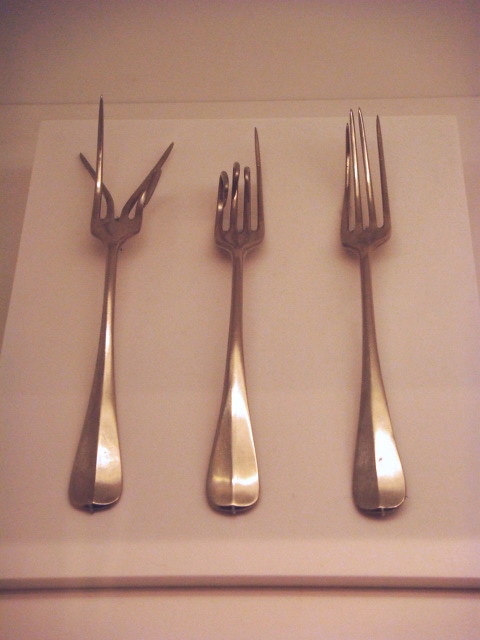This image showcases three artistic forks placed side by side on a beige napkin. Each fork is unique, featuring four tines that have been meticulously manipulated, giving the composition a distinct, sculptural quality. The leftmost fork has an intricate pattern where two of its tines are twisted, with one bent underneath. Its overall appearance is dynamic, as if the tines are engaging in a delicate dance. The middle fork also has a captivating structure, with its four tines varying in length—short, long, short, and the longest—suggesting a functional yet whimsical design, almost as if the longest tine is poised to spear an object. The rightmost fork, simpler yet equally compelling, has its middle tines pressed closely together while one is slightly bent upward and to the left. The entire image carries a brownish tint, enhancing the warm and elegant feel of the scene.